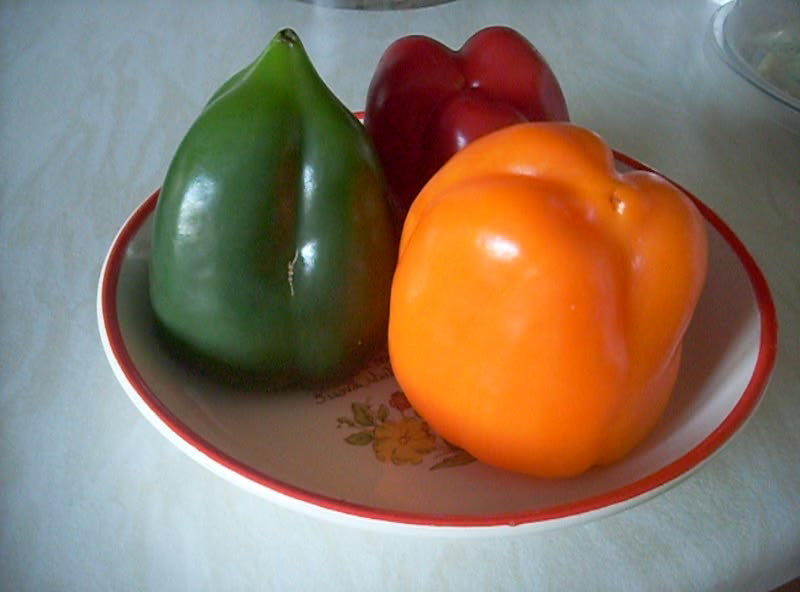This image showcases a close-up perspective of three vibrant bell peppers arranged on a small white plate adorned with a floral design and a red rim. The green pepper is positioned in the left back, the orange pepper, which appears the largest, sits prominently in the foreground, and the red pepper is slightly tucked behind the orange one, adjacent to the green pepper. The plate is set on a white tablecloth, and in the top right-hand corner of the image, a glimpse of transparent glass crockery, possibly a lid or a bowl, is partially visible. The floral pattern on the plate includes yellow and red flowers with green leaves, adding a delicate decorative touch to the scene. The lighting casts gentle reflections, enhancing the vivid colors of the peppers and the intricate details of the plate.